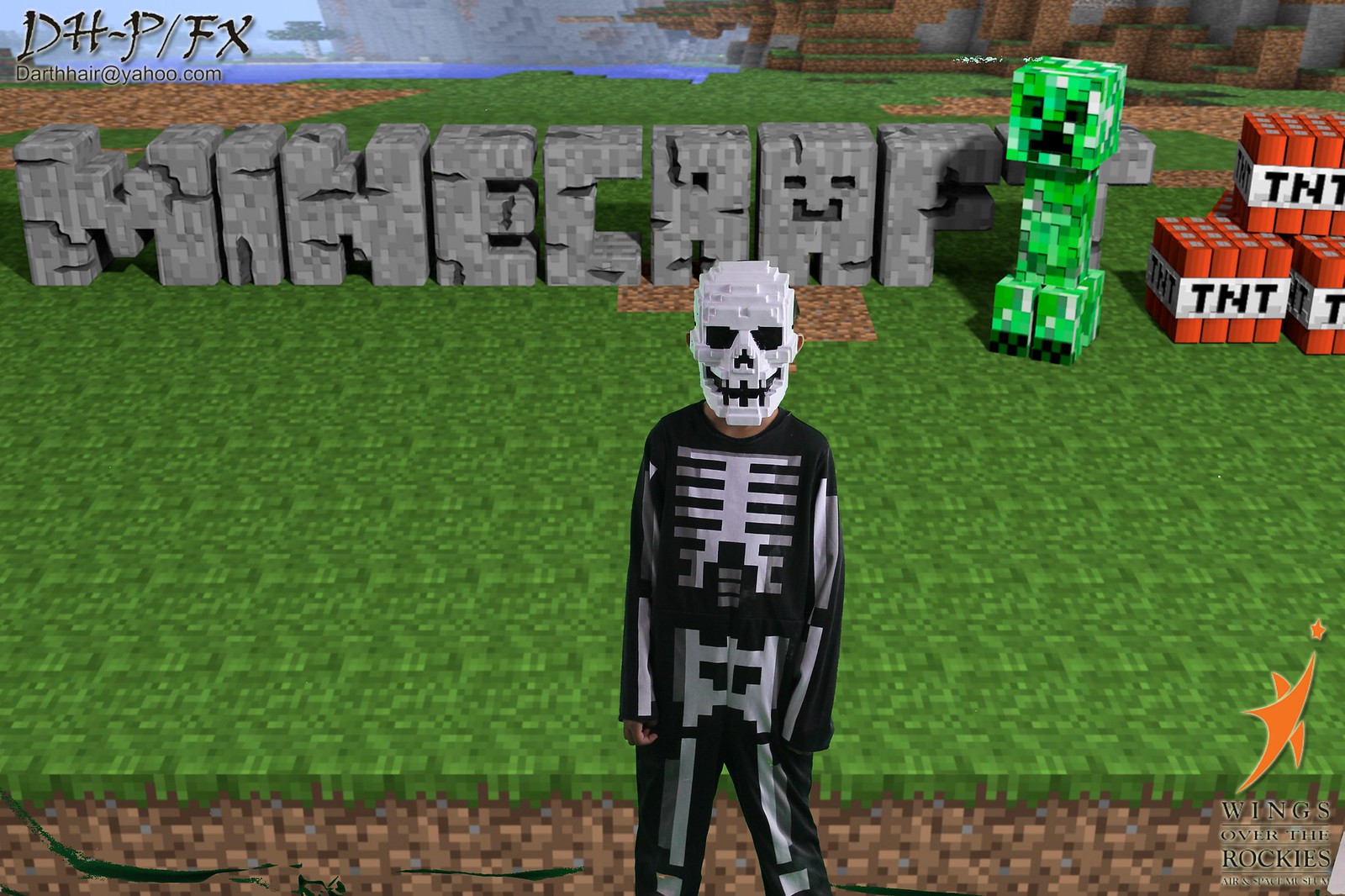The image is a computer-generated snapshot from the video game Minecraft, showcasing a Halloween-themed version of the game. Prominently featured is a character in a black outfit adorned with a white skeleton pattern, topped with a blocky skull mask, staring directly at the viewer. The Minecraft logo, in large gray block letters, stretches across the upper part of the image, seemingly growing out of a grassy ground. The backdrop includes an array of red, cube-shaped TNT blocks labeled "TNT," partially visible behind the character. There's a distinctive green figure with a rectangular face and thin body structure in the background. Additional elements include a scenic mix of snowy mountains, water, ocean, and clouds, creating a dynamic, detailed landscape. The upper left corner bears the text "dh-p/fx.air@yahoo.com" in black letters. The lower-right corner displays the logo for the "Wings Over the Rockies Air and Space Museum" with some illegible text beneath. The image conveys a playful, blocky aesthetic reminiscent of Lego figures, combined with classic Halloween costume elements.